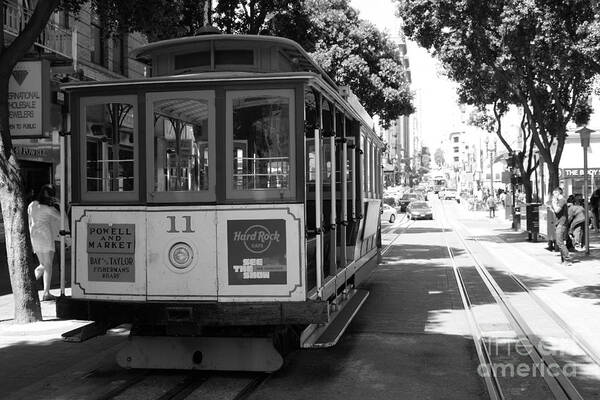This black and white photograph captures a vintage San Francisco trolley car, identified by the "Powell and Market" sign on its left side and an advertisement for the Hard Rock Cafe on its right. The trolley, marked with the number 11 and featuring a center light beneath three back windows, lacks visible passengers or a conductor, suggesting it may be parked. Decorative paneling and hand railings accentuate its classic design. The trolley rails are embedded in the street, suggesting it's ready for transit. The scene includes modern cars in the background, emphasizing its contemporary setting. The streets are lined with tall buildings and leafy trees, with pedestrians and another distant trolley adding to the lively urban environment. Overlay text "The Art America" is partially transparent in the bottom right corner, subtly branding the image.